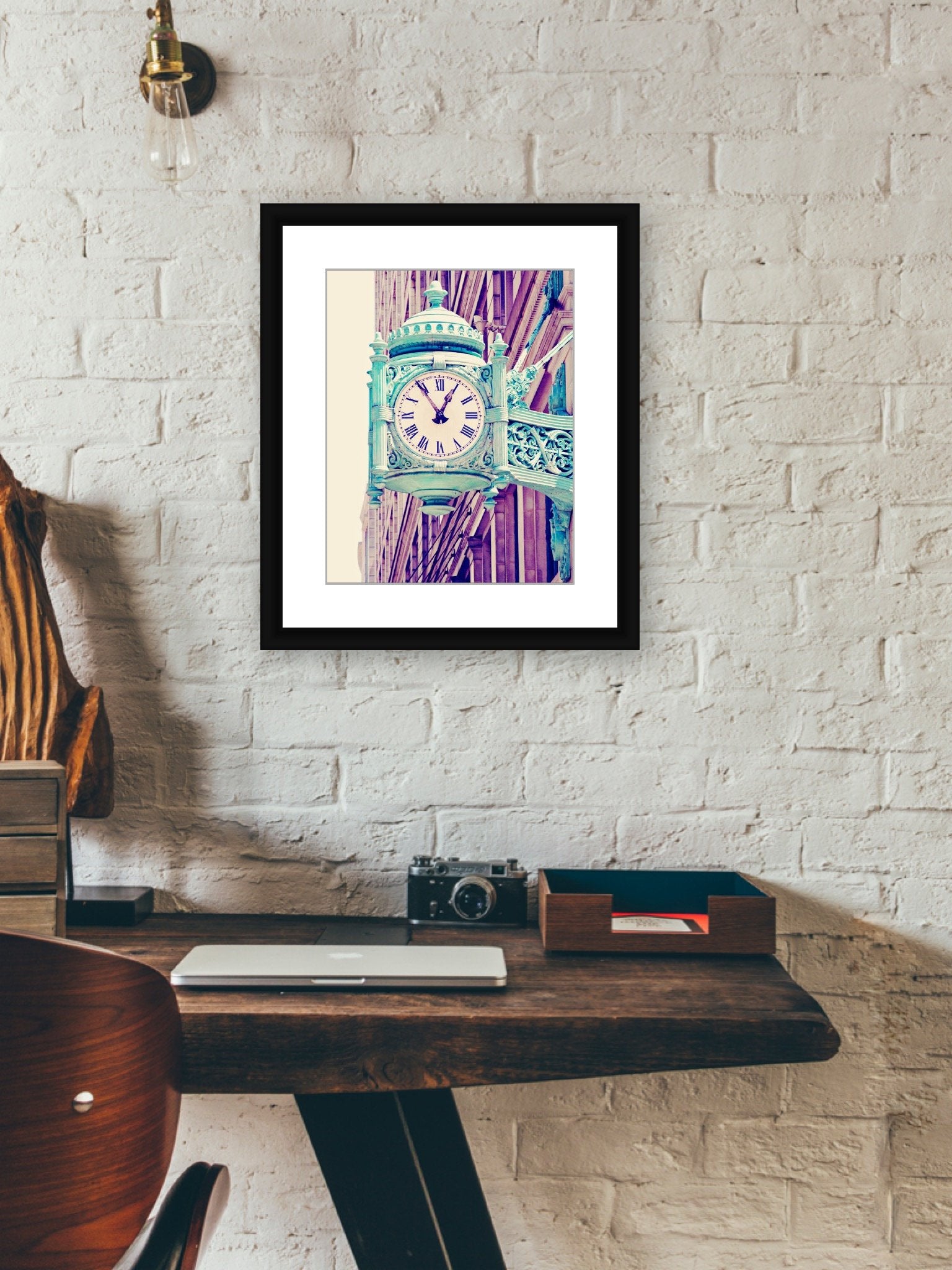The photograph showcases an evocative art piece displayed on a white brick wall that exudes an organic, imperfect charm. Adding to the character of the scene, a brass lamp with a distinct steampunk aesthetic is mounted in the upper left corner of the wall. The lamp, featuring a single oversized clear bulb, complements the eclectic atmosphere of the setting.

Centrally framed within the image, a black-framed art piece with a white border captures attention. The artwork depicts a teal-colored clock tower displaying the time 12:55, with Roman numerals adorning its face. Behind the clock tower, a contrasting pink building adds depth and intrigue to the composition.

Beneath this framed art piece, the image captures the edge of a rustic, dark wooden desk with slightly burnt edges, epitomizing a raw, natural elegance. On the desk rests an assortment of items, including a vintage camera, a paper tray, and a closed laptop, all contributing to a nostalgic yet functional office setup. The desk, supported by mid-century modern legs that angle out diagonally, further enhances the stylistic fusion. To the right, the back of a modern office chair with a wooden frame partially peeks into the frame, suggesting a cohesive blend of contemporary and vintage elements in the workspace.